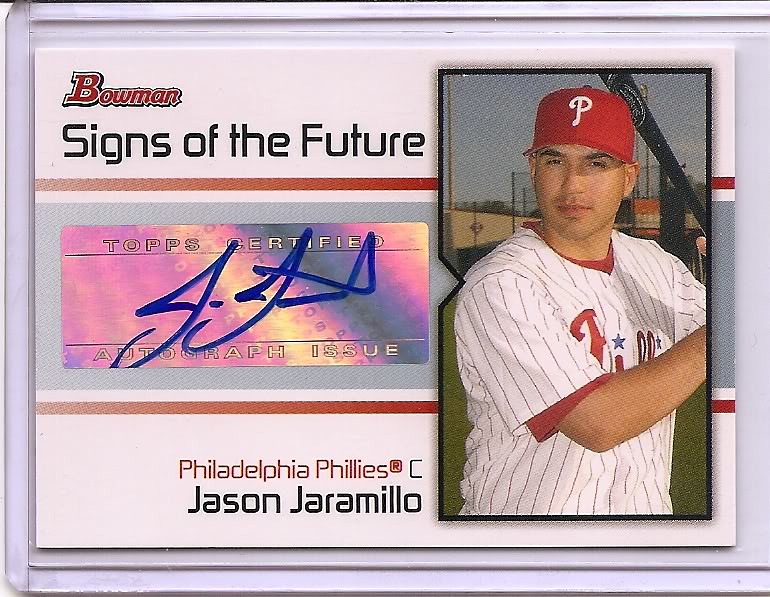Encased in a protective plastic cover, the baseball card features a dynamic photograph of Philadelphia Phillies catcher Jason Jaramillo. He is poised as a left-handed hitter, gripping a black bat, dressed in a white pinstriped jersey over a red short-sleeved shirt, and a matching red cap emblazoned with the Phillies' emblem. Against a backdrop of a baseball field fence and wall, the card exudes a sense of authenticity and pride. The top portion of the card showcases the bold red "Bowman" logo with a slight pink background, accompanied by the black text "Signs of the Future." Adding to its collectability is the metallic, glossy "TOPS Certified Autograph Issue" sticker in the gray section, bearing Jaramillo's blue-ink signature. At the bottom of the card, "Philadelphia Phillies, C. Jason Jaramillo" is prominently printed in red, cementing its status as a collector's item.